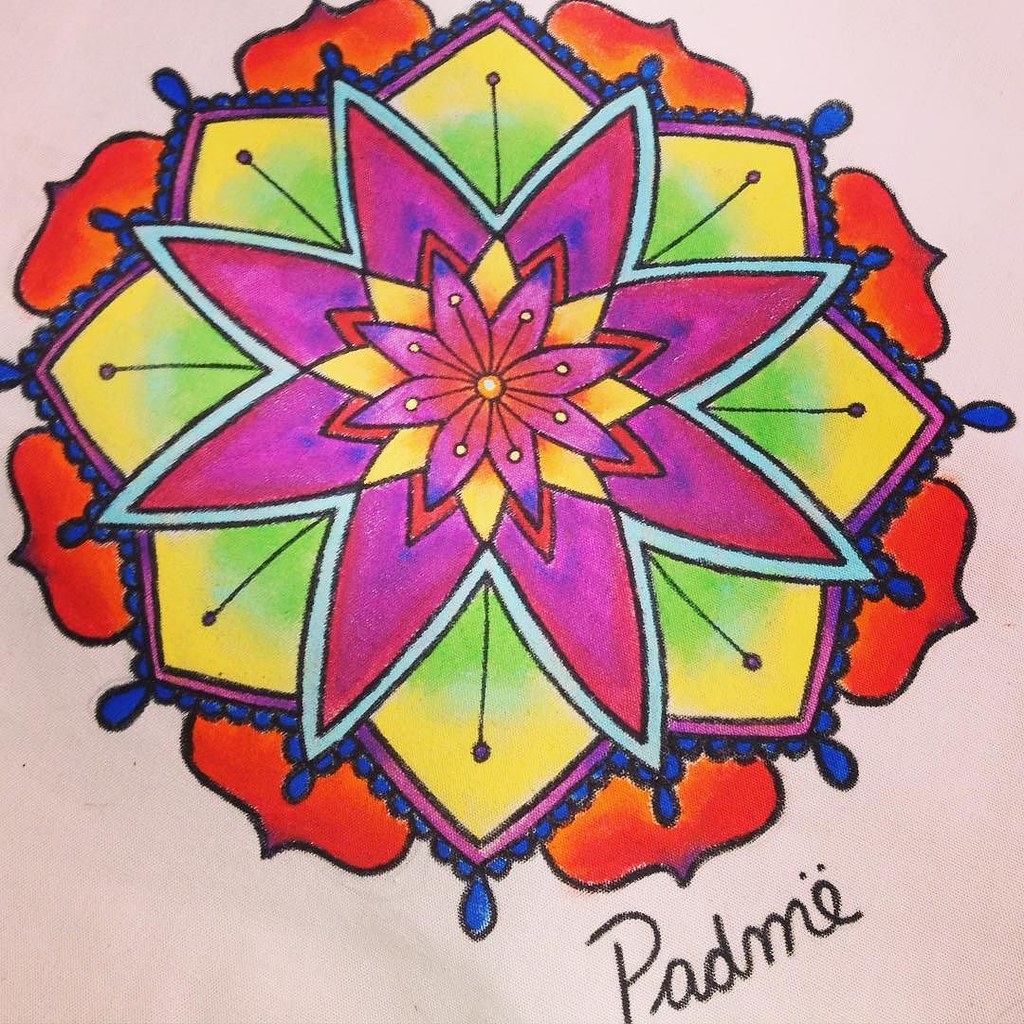The image is a detailed and vibrant digital artwork of a multi-layered, star-shaped flower with six layers of petals. At the very center is a pink core with orangish and yellow pollen. Surrounding this core are pink petals edged with purple tips, adorned with yellow pollen-like dots and intricate lines. Just beyond, another flower's yellow petals with an orange center peek through. Further out, there are orange petals interlaced with purple ones. These layers are framed by a larger purple and pink flower featuring red detailing on each petal, and blue accents within the interior spaces. This is all encompassed by a teal outline and ensconced in a yellowish-green outer flower, which transitions to a yellow edge. This outer layer is bordered by a pink rim and completed with a scalloped blue edge. Behind this vibrant composition is another reddish-orangish flower set against an off-white background. In the bottom right corner, the artist's signature "Padme" is inscribed in black script.